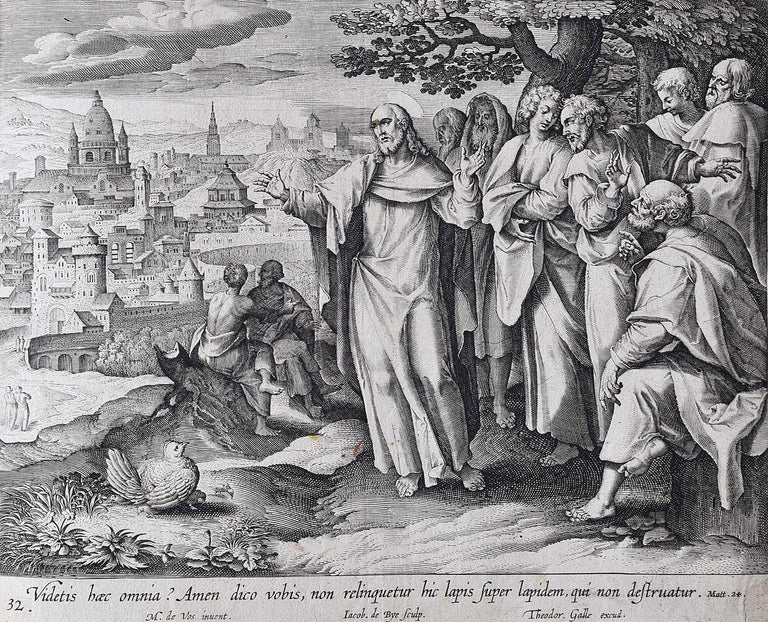This scanned black-and-white sketch, likely a reproduction of an older artwork, depicts a religious scene centered around Jesus Christ. He stands barefoot in long robes with a halo above his head, raising both hands as if speaking. Surrounding him are nine or ten figures in classical Roman dress, indicative of a Biblical scene. To the right, a group of men is engaged in conversation, with one bearded and hooded, and another bald. Two more individuals are shown seated to the left on a log. In the background, a classical cityscape with domes and temple-like structures is visible. A tree with leaves and some clouds add to the scene's atmosphere. Detail at the bottom includes text in Latin and the number 32 in the lower left corner. The only colors in the artwork are various shades of black and white, enhancing its classical and solemn tone. Additionally, a bird, possibly a chicken, looks up at Jesus from the left-hand side of the foreground.